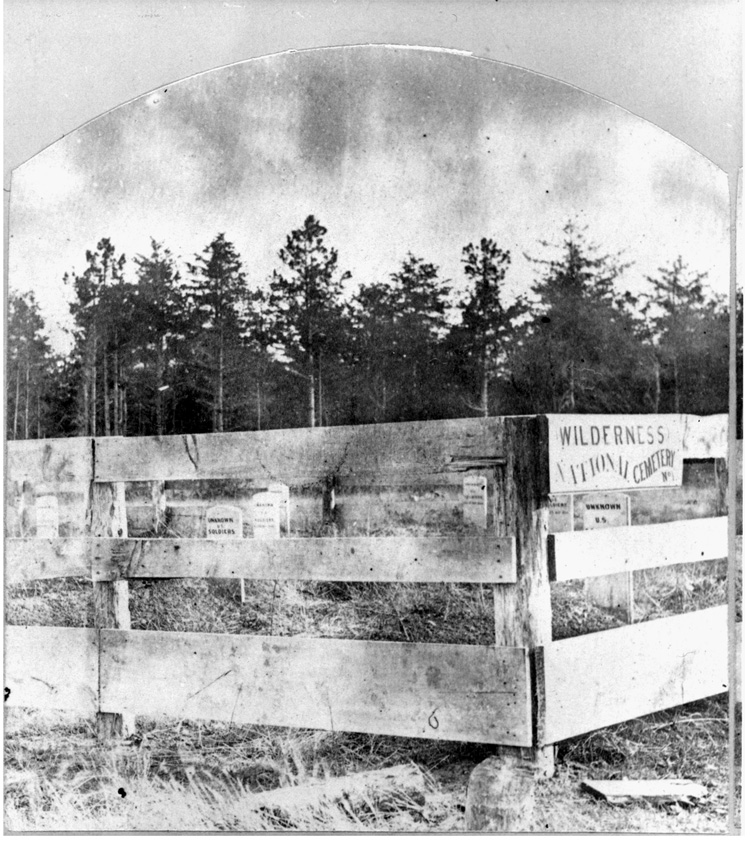This black and white photograph, likely from the 1800s, depicts the solemn scene of the Wilderness National Cemetery. The image is cut out in a circular shape with the top forming a half-oval. In the background, the sky appears gray and murky, possibly due to the vintage nature of the photograph, and it is framed by a dense forest with trees in varying shades of dark gray to black.

In the middle ground, a wooden fence constructed from three horizontal slats – a thicker one at the bottom, a middle one, and a thinner top slat – borders the cemetery. An inscription on the fence reads "Wilderness National Cemetery." Between the fence slats, numerous tombstones are visible, nestled among the forested area, adding to the somber atmosphere.

In the foreground, there is a scattering of wood pieces and rocks, potentially debris from the cemetery. The grass seems dead or barren, enhancing the melancholy tone of the scene. The border of the image reveals a glimpse of another photo placed beside it on what appears to be an old backdrop, enhancing the historic feel of the captured moment.